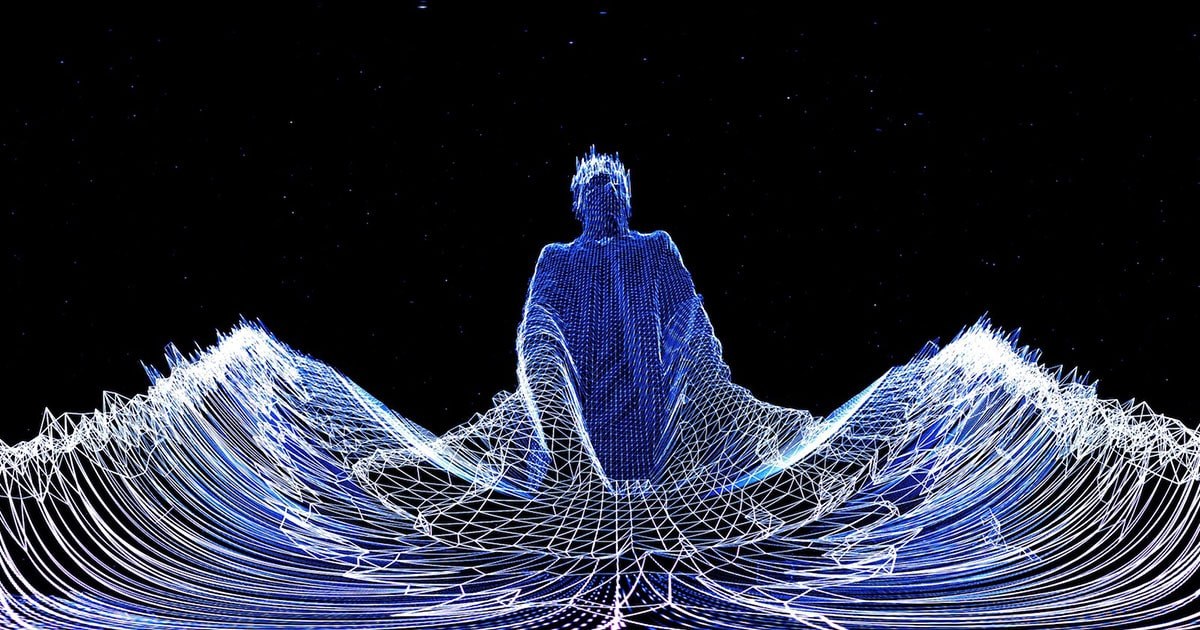This digitally rendered image portrays a figure composed of blue and white pixels emerging from the midst of sound waves. The man, depicted in a checkerboard pattern of blue-tinted squares, seems to rise from an abstract, star-studded black background. His form, defined by a distinctive blue hue and contrasting white accents, appears to be extending his arms outward, parting large sound waves on either side. These waves are illustrated by flowing white and blue lines that traverse the entirety of the composition. Intricate details, such as a white cap that resembles a crown possibly due to reflections and his fully covered, long outfit, add to the surreal and contemporary aesthetic of the piece. The vibrant blue and white visuals stand out starkly against the black expanse, enhancing the intriguing and modern feel of the image.